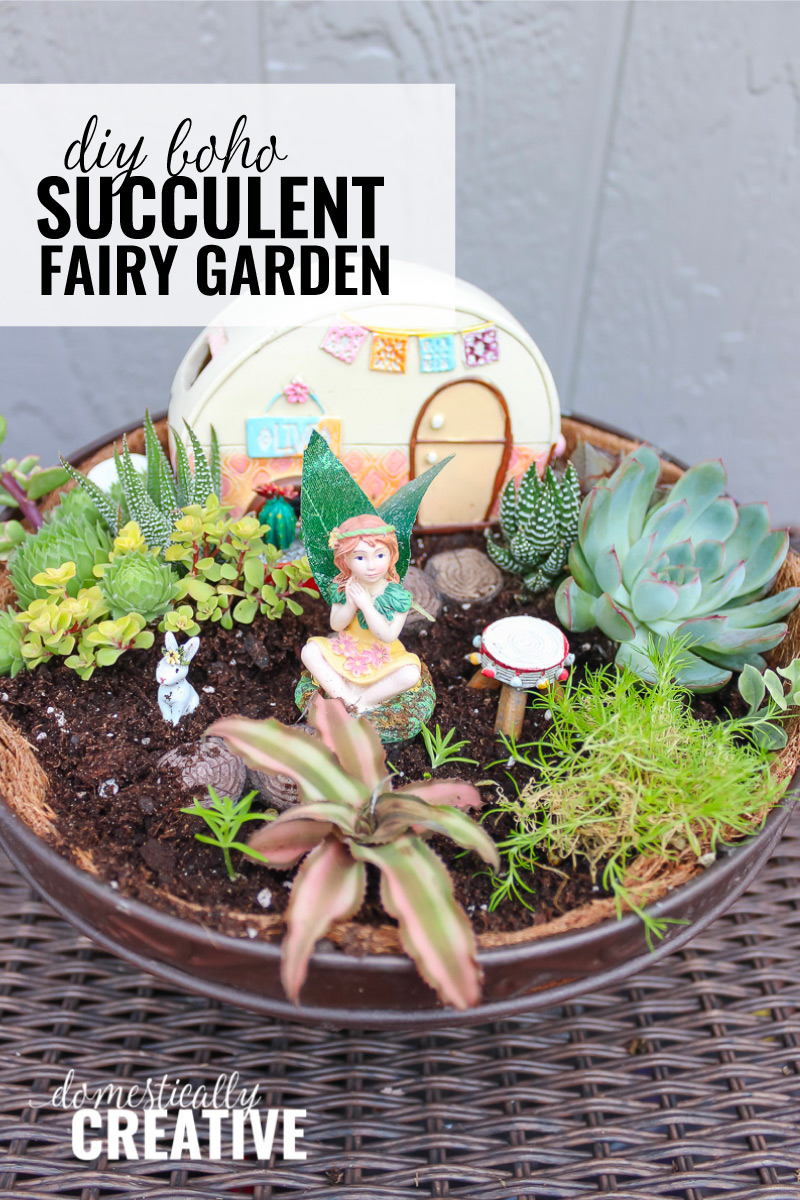This image depicts the first page of an instructional booklet for creating a DIY Boho Succulent Fairy Garden. The centerpiece of this tiny garden is a round, ceramic brown bowl filled with soil, showcasing an assortment of succulents, including varieties like aloe and hens and chicks, primarily in shades of green, with one featuring red streaks. At the heart of this miniature landscape sits a petite figurine of a red-haired fairy in a green and yellow dress, her legs crisscrossed as she perches likely on a green lily pad. Around her, a white bunny figurine adorned with a flower adds an extra touch of whimsy. Behind the fairy, a small model RV camper serves as a fairy house, adding to the charm of the scene. The garden appears to be displayed outdoors on a wicker table. Above the planter, text reads "DIY Boho Succulent Fairy Garden," emphasizing its bohemian style, while the bottom of the image is branded with "Domestically Creative," presumably the sponsoring company.